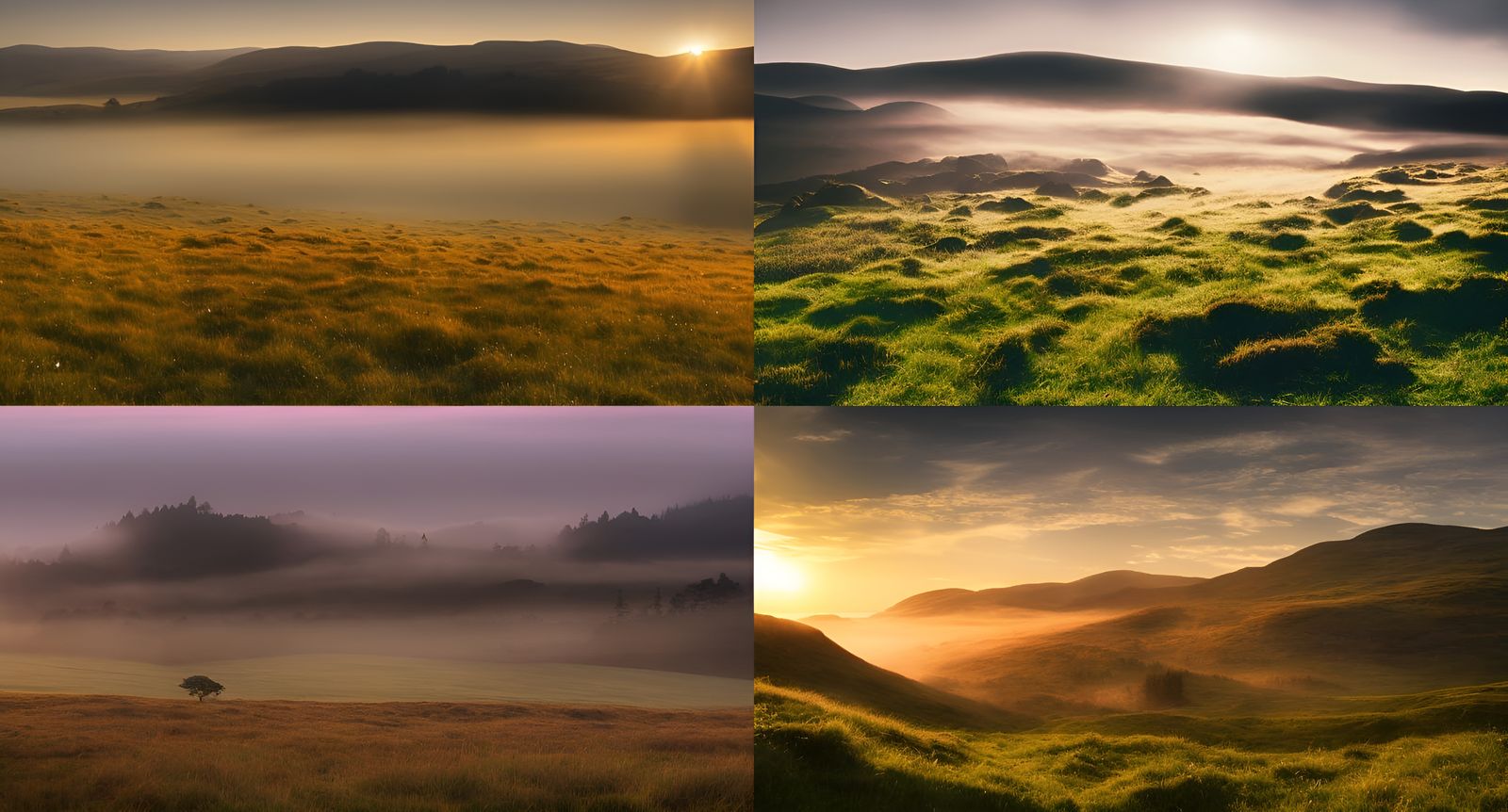This image comprises four distinct landscape photographs, each capturing serene natural scenes with mountains, grasslands, and fog under varying conditions of sunrise or sunset. In the upper left, a misty landscape with brownish grass suggests a winter or fall setting, with the sun rising behind distant mountains. The upper right shows a more vibrant scene with lush green grass and a sunrise illuminating the mountains. The bottom left features rolling hills and fog, with lifeless, brown grass under a gray sky. The bottom right displays a lush green valley, where the sunrise meets light clouds, offering a refreshing contrast to the more muted tones of the other images. Each photograph shares common elements of mountains, grasslands, and the sun's early light, yet they collectively highlight the diversity and beauty of natural landscapes through different seasons and times of day.